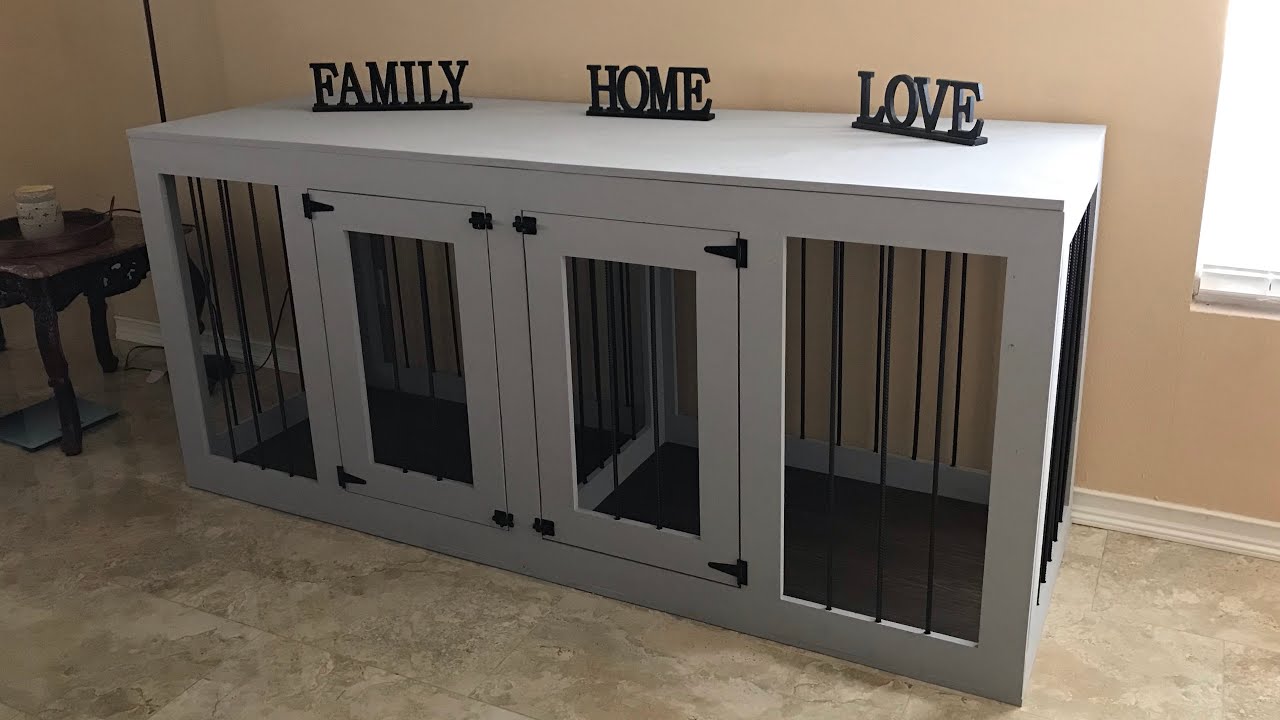This photograph showcases a scene inside a home, featuring a large, rectangular piece of furniture that serves as a dog crate. The dog crate, which is light gray or silver in color, is positioned on a beige and gray marbled tile floor against a light peach or tan wall with white baseboards. The crate has two doors with a divider in the middle and thin black steel bars in front of the windows. To the left of the crate, there is a small brown side table holding an object. On top of the dog crate, three black plaques stand upright, each inscribed with the words "family," "home," and "love." Off to the right side of the image, a lone window is visible.